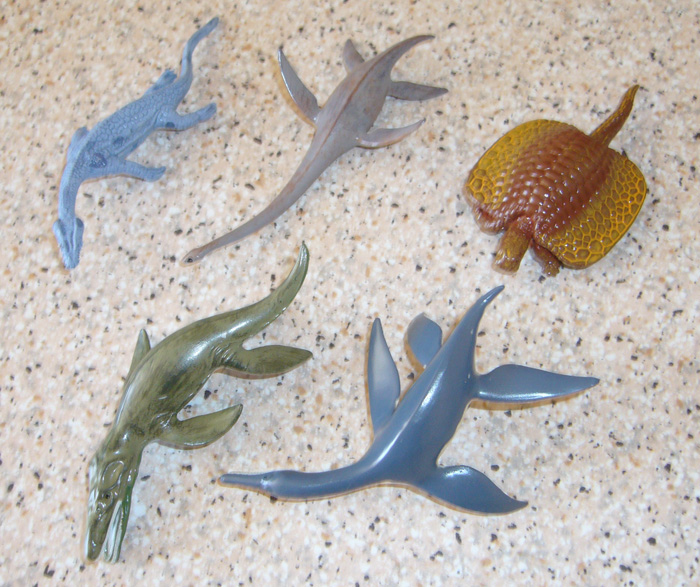This photograph, taken from a top-down perspective on a beige granite countertop flecked with black, white, and amber spots, showcases five realistic-looking toy figurines made of rubber or plastic, resembling ancient sea creatures. In the forefront on the right side, there's an orange squarish creature with a turtle-like head, dark brown center, yellow sides, and a long tail, somewhat resembling a stingray. Nearby on the left, a green porpoise-like toy with a long snout and teeth is visible, showing three of its flippers and a tail. Above this, on the right side, is a blue toy with four legs and a long neck. Next to it, a gray toy with a slender, snake-like neck and four flippers is placed. Lastly, in the upper left corner, there's another blue creature with four legs, an eel-like body, a snake head, and a long tail. These detailed figurines evoke the appearance of ancient sea dinosaurs and add a playful element to the speckled background.